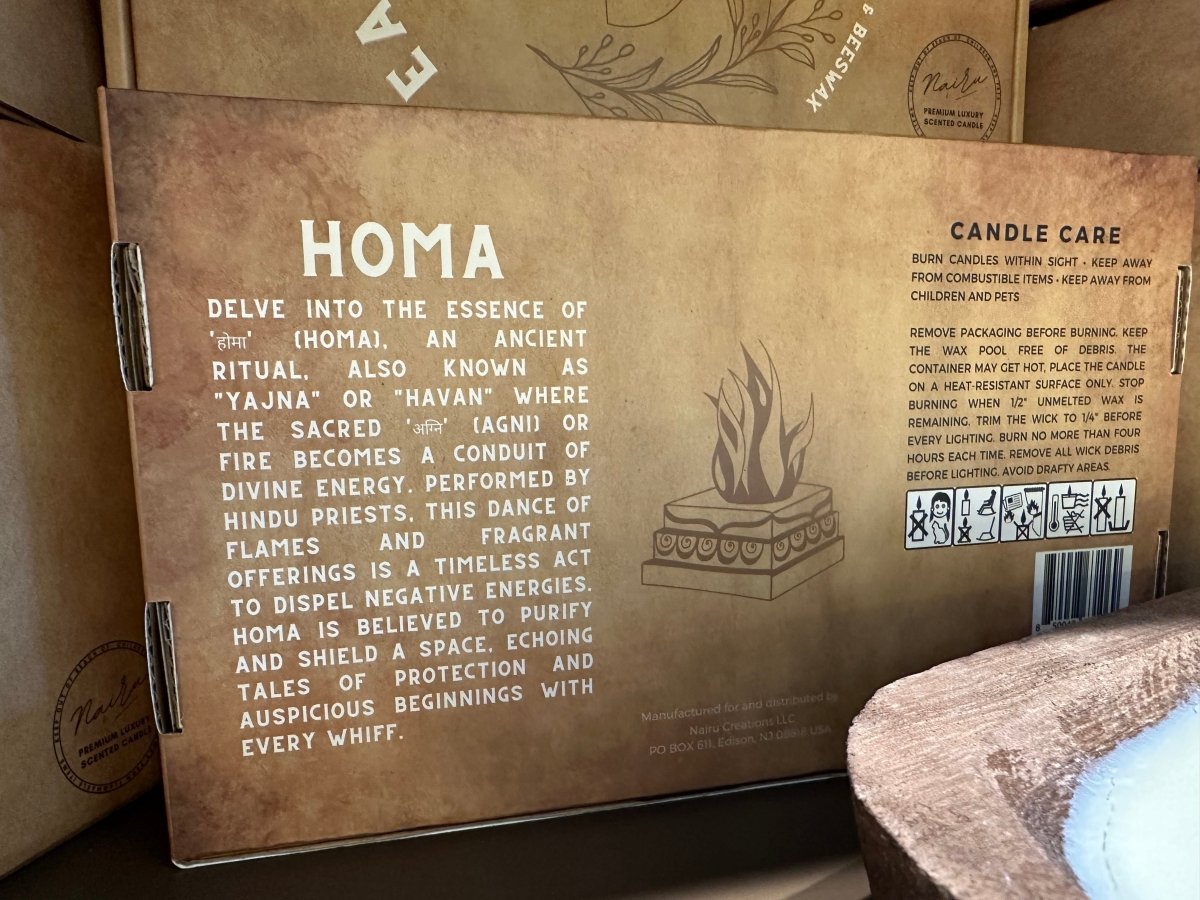The image displays the back of a worn, ancient-styled, brown cardboard box that holds a Homa candle, manufactured by Nara Creations, LLC. The box features an intricate illustration in the center showing a three-tiered base with a wax flame on top, symbolizing the candle itself. On the left side in white text, a detailed description reads: "Delve into the essence of Homa, an ancient ritual also known as Yajna or Havan, where the sacred Agni, or fire, becomes a conduit of divine energy performed by Hindu priests. This dance of flames and fragrant offerings is a timeless act to dispel negative energies. Homa is believed to purify and shield a space, echoing tales of protection and auspicious beginnings with every whiff."

On the right side, black text provides comprehensive candle care instructions: "Burn candles within sight. Keep away from combustible items, children, and pets. Remove packaging before burning. Keep the wax pool free of debris. The container may get hot; place the candle on a heat-resistant surface. Only stop burning when half-inch unmelted wax is remaining. Trim the wick to 1/4 inch before every lighting. Burn no more than four hours each time, removing all wick debris before lighting. Avoid drafty areas." The packaging also includes cautionary images representing these guidelines to ensure safe usage.